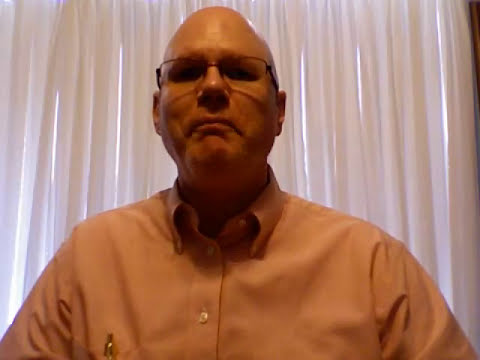The image features a middle-aged, bald Caucasian man, possibly in his mid to late 30s. He is wearing eyeglasses and an off-white long-sleeved button-down shirt with a collar. The shirt is neatly buttoned, and a gold-tipped pen is tucked into a pocket on the left side of his chest. His expression is solemn and somewhat somber as he looks slightly downwards towards the camera, suggesting he may be participating in a video call. He is positioned in a room with white curtains behind him, through which daylight streams, casting soft light patches. The setting could be a hotel room, given the typical white curtains and the overall ambiance.